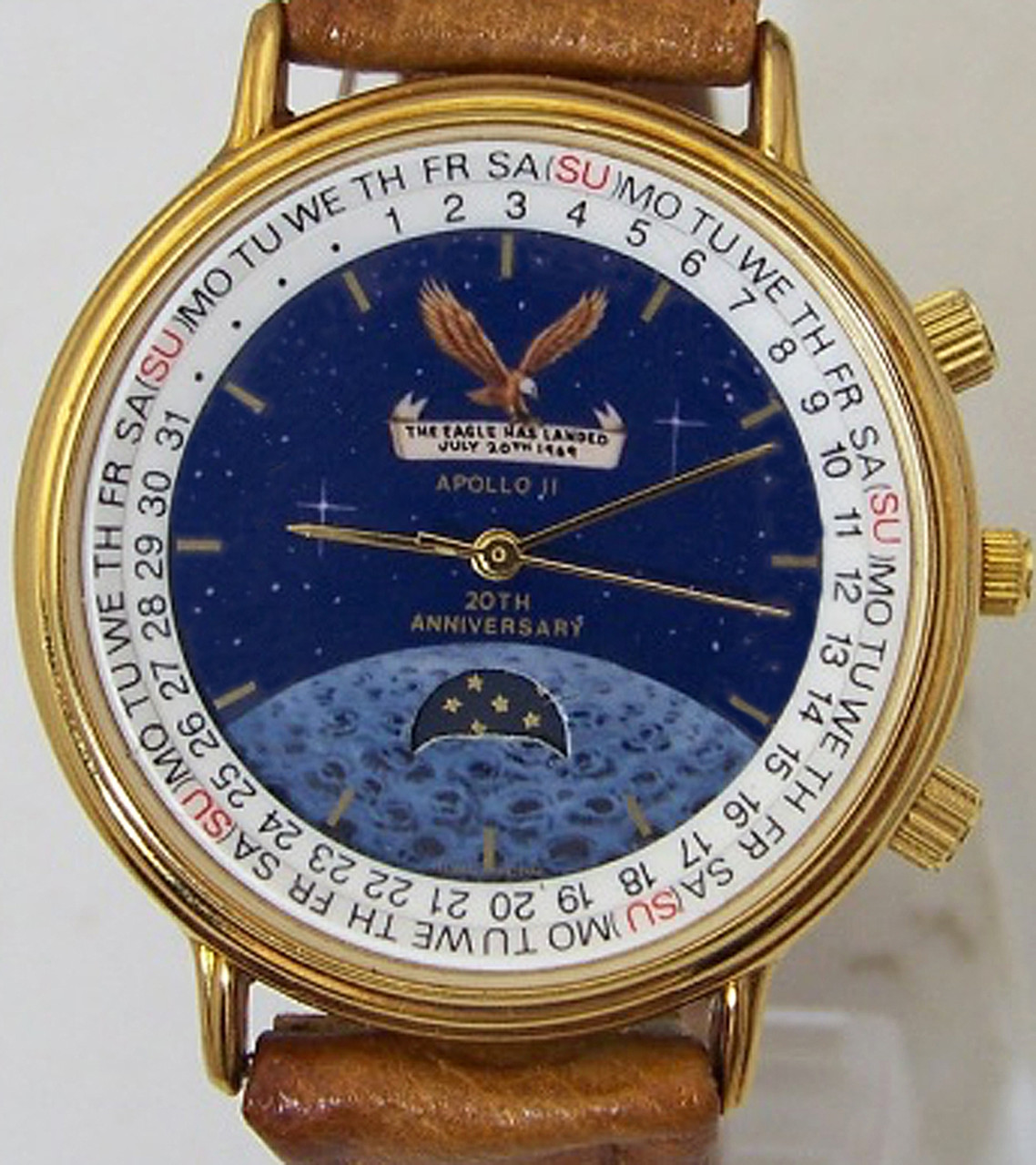This detailed image presents a close-up view of an elegant wristwatch with a light brown leather band and gold accents around its large, circular face. Set against a white background, the watch is the focal point of the photograph. The watch face features an intricate design: an eagle in mid-flight at the top, with wings spread wide. Below the eagle is the inscription, "The Eagle Has Landed, July 20th, 1969," commemorating the Apollo 11 moon landing. The text "Apollo 11" appears just beneath this inscription. The background of the watch face is a deep blue, dotted with stars and a depiction of the moon's surface. The watch hands display a time around 9:12, with the second hand between the 12 and 13. Gold lettering below the hands reads "20th Anniversary." Additionally, the watch includes a detailed outer ring, listing the days of the week, Monday through Sunday, and the days of the month, 1 through 31. The attention to detail and elegant design make this watch a notable commemorative piece.